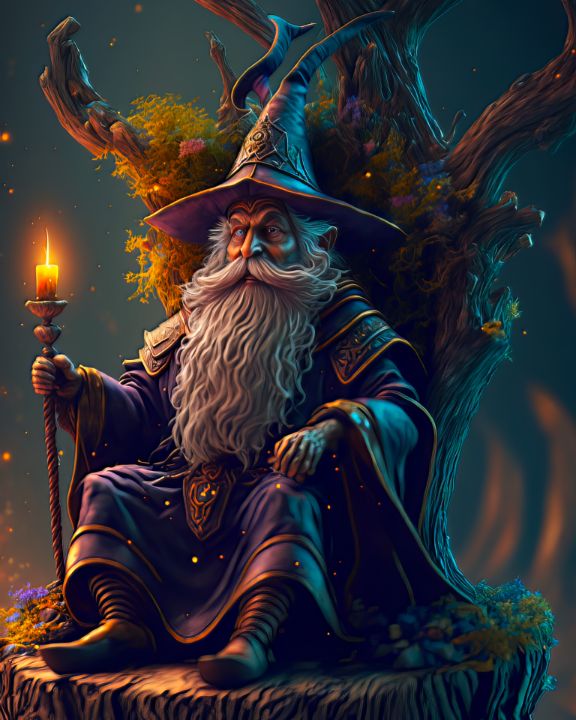This detailed digital illustration depicts an elderly wizard seated on a grand, throne-like structure formed from a twisted, fossilized tree. Adorned in a dark purple robe with intricate orange designs and long, flowing sleeves that almost reach the ground, the wizard cuts an imposing figure. His tall, pointed hat, similarly dark purple but with earthy brown hues, perches atop his head. His distinctive facial features include a pronounced nose, thick eyebrows, and high cheekbones, all framed by a flowing, wavy gray beard and a large mustache.

The wizard's right hand clutches a staff crowned with a burning candle, casting a warm, flickering light that contrasts with the dark, star-dotted sky in the background. His left hand calmly rests on the arm of his arboreal throne, his feet stretched out and clad in pointed, metallic-hued boots. The tree throne itself has branches extending upwards and is adorned with occasional patches of moss and delicate pink flowers, adding a touch of nature's beauty to the mystical scene.